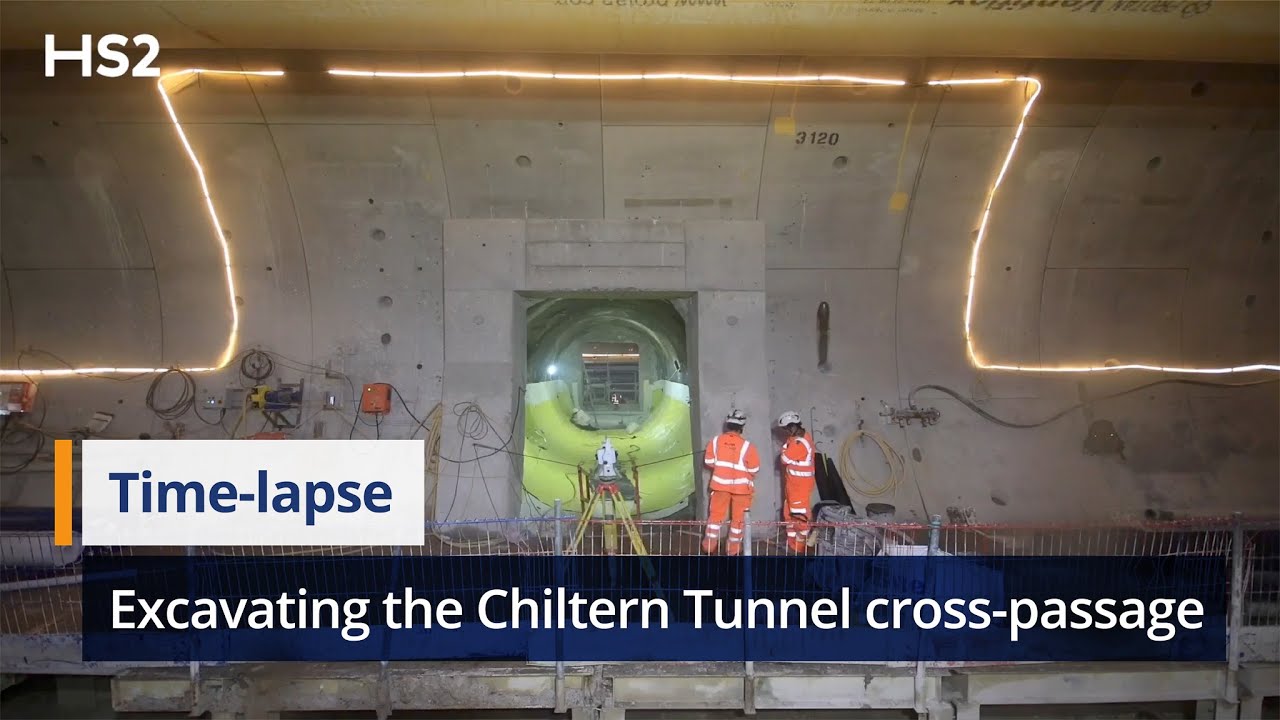This image is likely a screenshot from a news channel or YouTube video. It depicts an underground scene, specifically the excavation of the Chiltern Tunnel cross passage, as indicated by the text overlay. On the top left, the label "HS2" is visible. At the bottom, text in a white rectangle with blue font reads "time-lapse," and below that, in a longer blue rectangle with white font, it says "excavating the Chiltern Tunnel cross passage."

The scene is set in a concrete tunnel, which branches into another tunnel extending into the horizon. The second tunnel's floor is painted orange or yellow. Two men in bright orange, high-visibility suits with reflective stripes and hard hats stand on a platform next to the entrance of this secondary tunnel. They are looking down the tunnel, with a variety of construction tools surrounding them. The primary tunnel is illuminated by a series of lights running from left to right, highlighting its concrete structure and the numerous wires and construction materials present.